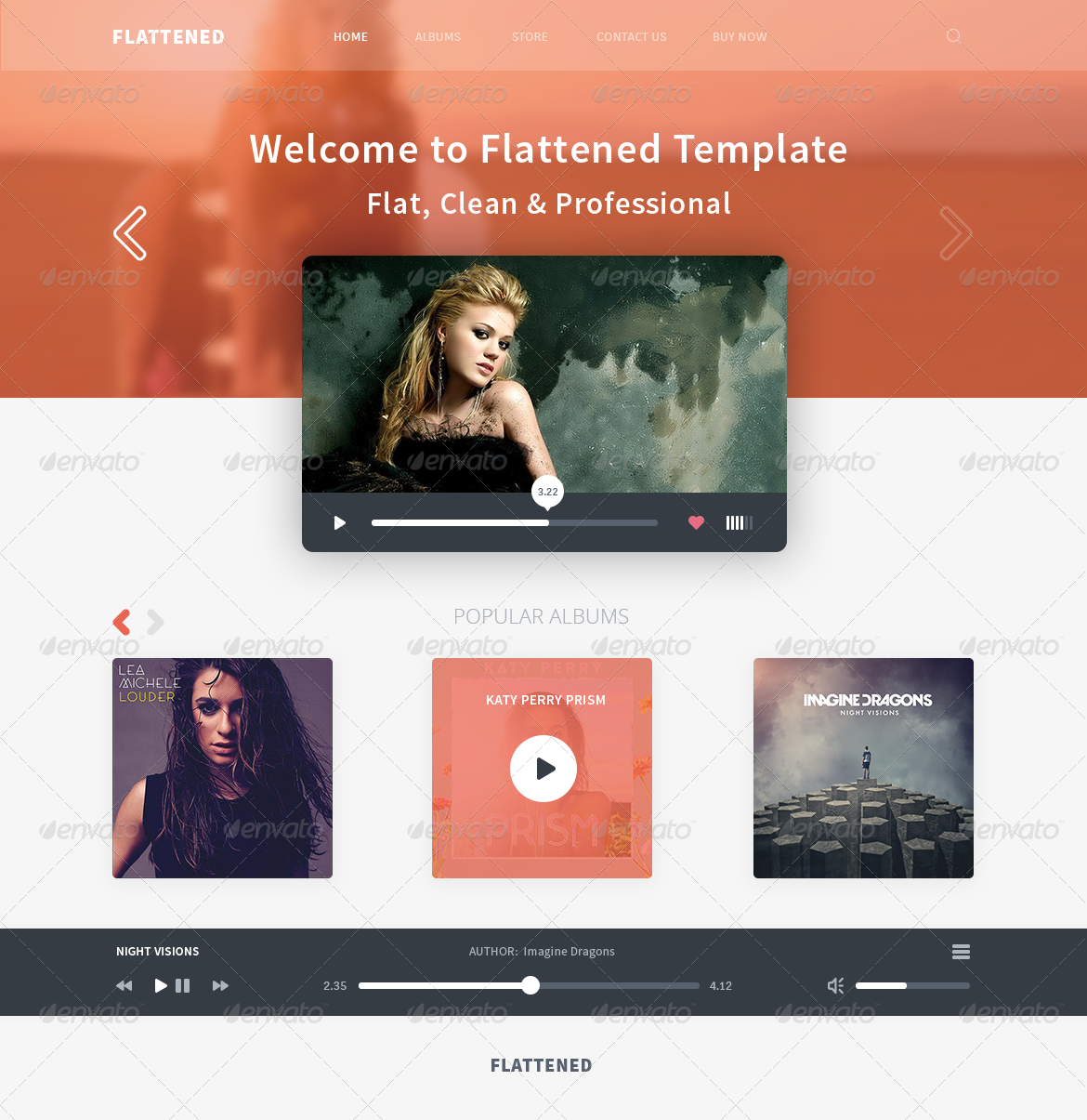This image is a detailed screenshot of a website template. At the very top, the background consists of subtly blended shades of pink and orange, resembling a panoramic shot of nature. Faintly, a person's image can be discerned within the background.

The header features the word "FLATTENED" in bold, white capital letters. Below this, there's a menu, but the fonts are too light to be legible. Centrally, the prominent headline reads, "Welcome to a Flattened Template," followed by the tagline, "Flat, Clean, and Professional."

Beneath the headline, there's a square video player with a gray control bar at the bottom. The video showcases a Caucasian woman with long blonde hair, wearing a strapless black top reminiscent of a bodice.

The section below the video features a white background and displays three square images, which appear to be album covers. The first image on the left shows a white woman with dark hair partially covering her left eye, wearing a black sleeveless shirt. The middle image, set against a pink background, simply bears the title "Katy Perry - Prism." The third image on the right has a gray background with the band's name, "Imagine Dragons," displayed in white text.

At the very bottom, there is a media player with controls in varying shades of gray and white.